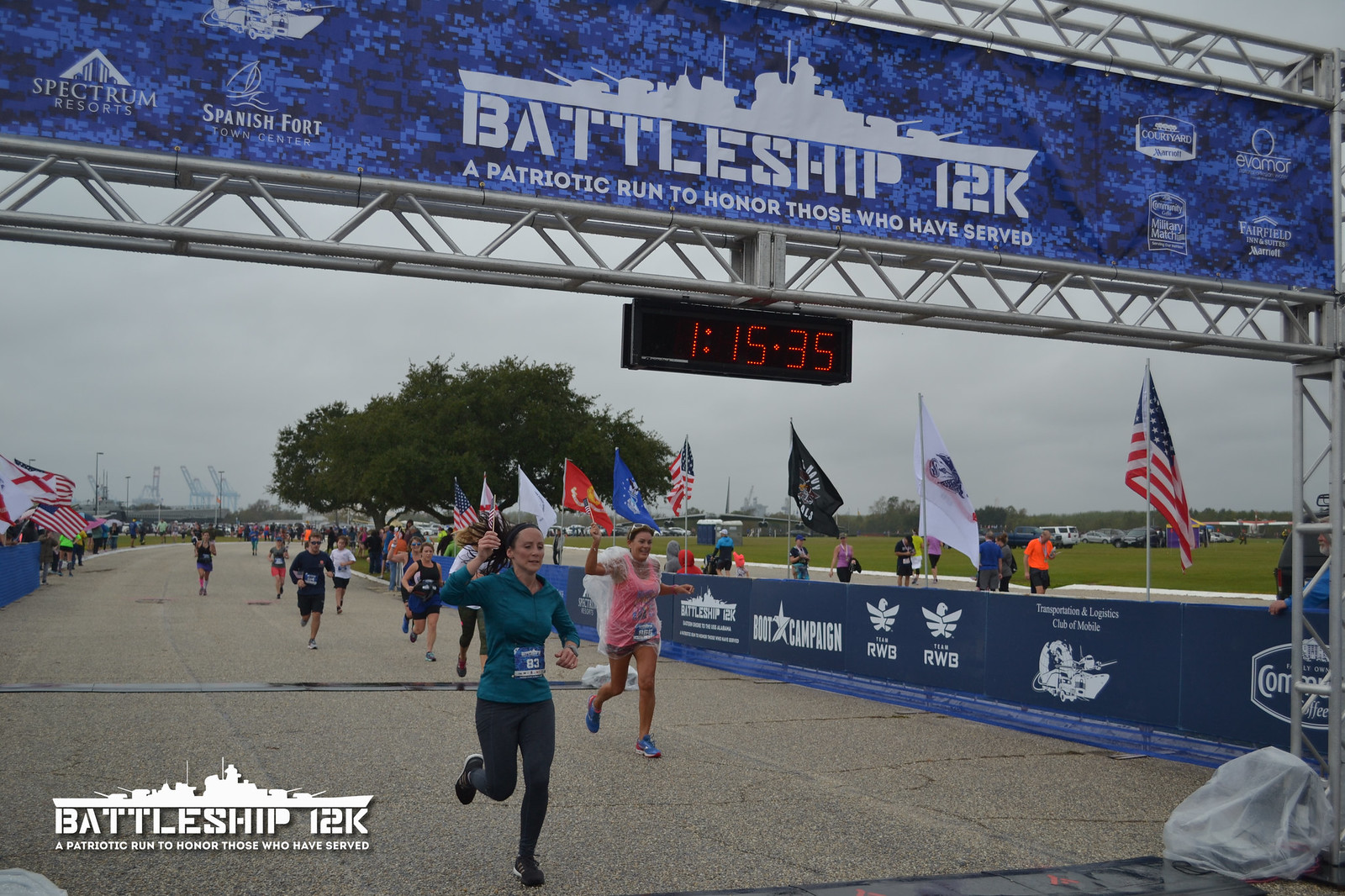The image captures the climactic moment at the finish line of the Battleship 12k, a patriotic run to honor those who have served. Dominating the upper section of the photo is a rectangular banner with a custom white-font "Battleship 12K" and a silhouette of a battleship, set against a blue background. The banner also features logos of sponsors who likely supported the event. Below the banner, a red LED timer displays "1:15:35," presumably showing the current elapsed time of the race. In the foreground, several runners are about to cross the finish line, with the two most prominent athletes being a person in dark green long sleeves and dark grey pants on the left, and another in a pink shirt, shorts, and blue and pink shoes on the right. The race track is flanked by flags and scattered spectators, some of whom appear to be casually walking rather than intently watching the event. A watermark in the bottom left corner repeats the event's name and purpose, "Battleship 12K, a patriotic run to honor those who have served," along with a small white battleship silhouette.